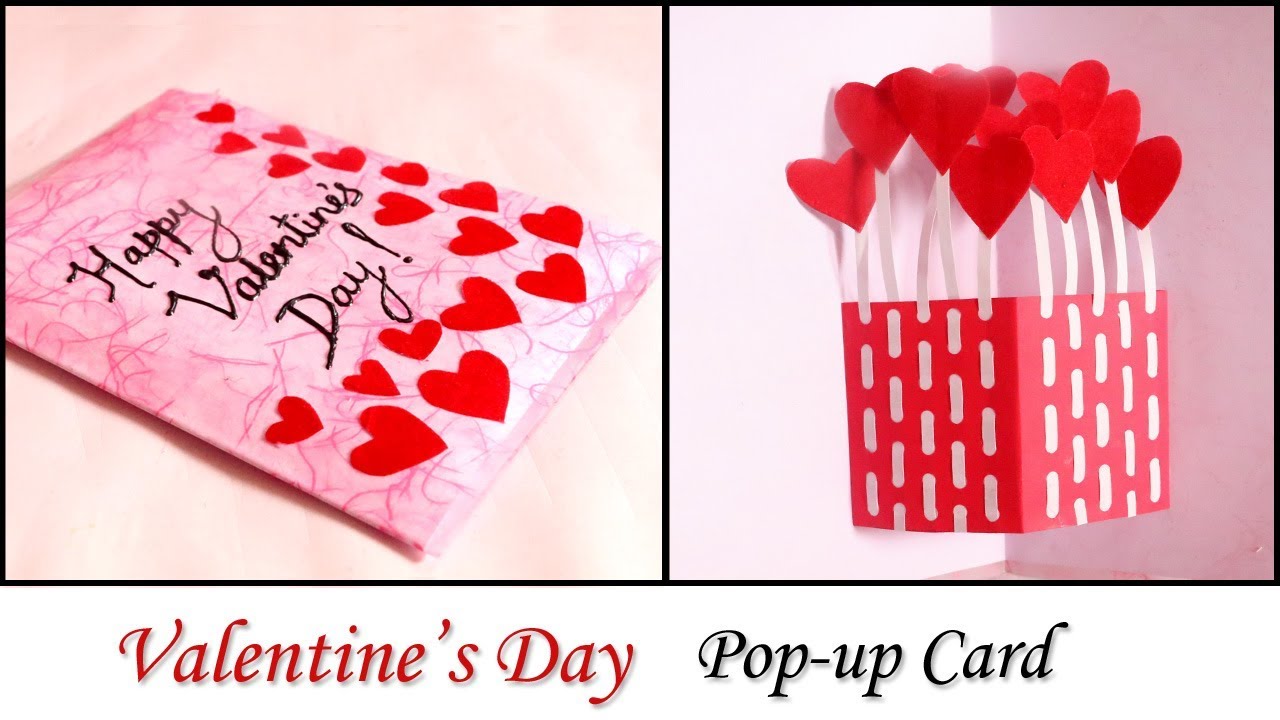The image features two side-by-side photos encased in a thin black border. On the left, there's a greeting card laying on a light pink surface. The card is a shade of pink with a marbled background and adorned with red hearts along its bottom and right edges. It is tilted counterclockwise about 60 degrees. "Happy Valentine's Day" is written in black, cursive, puff paint, adding a handmade touch to the card's front. Below this greeting, there's a red label that reads "Valentine's Day" in matching script font. 

To the right, the second photo displays the same card in an open position. The interior features a red pop-up design with vertical white lines, resembling a multi-storied building. White strips of paper extend upwards from the card’s top, each ending in either a red or white heart, totaling around ten in number. The detailing here meticulously captures the intricate, 3D elements of the pop-up card. Under these photos, in a white space, the text "Valentine's Day Pop-Up Card" is prominently displayed, with "Valentine's Day" in red and "Pop-Up Card" in black.